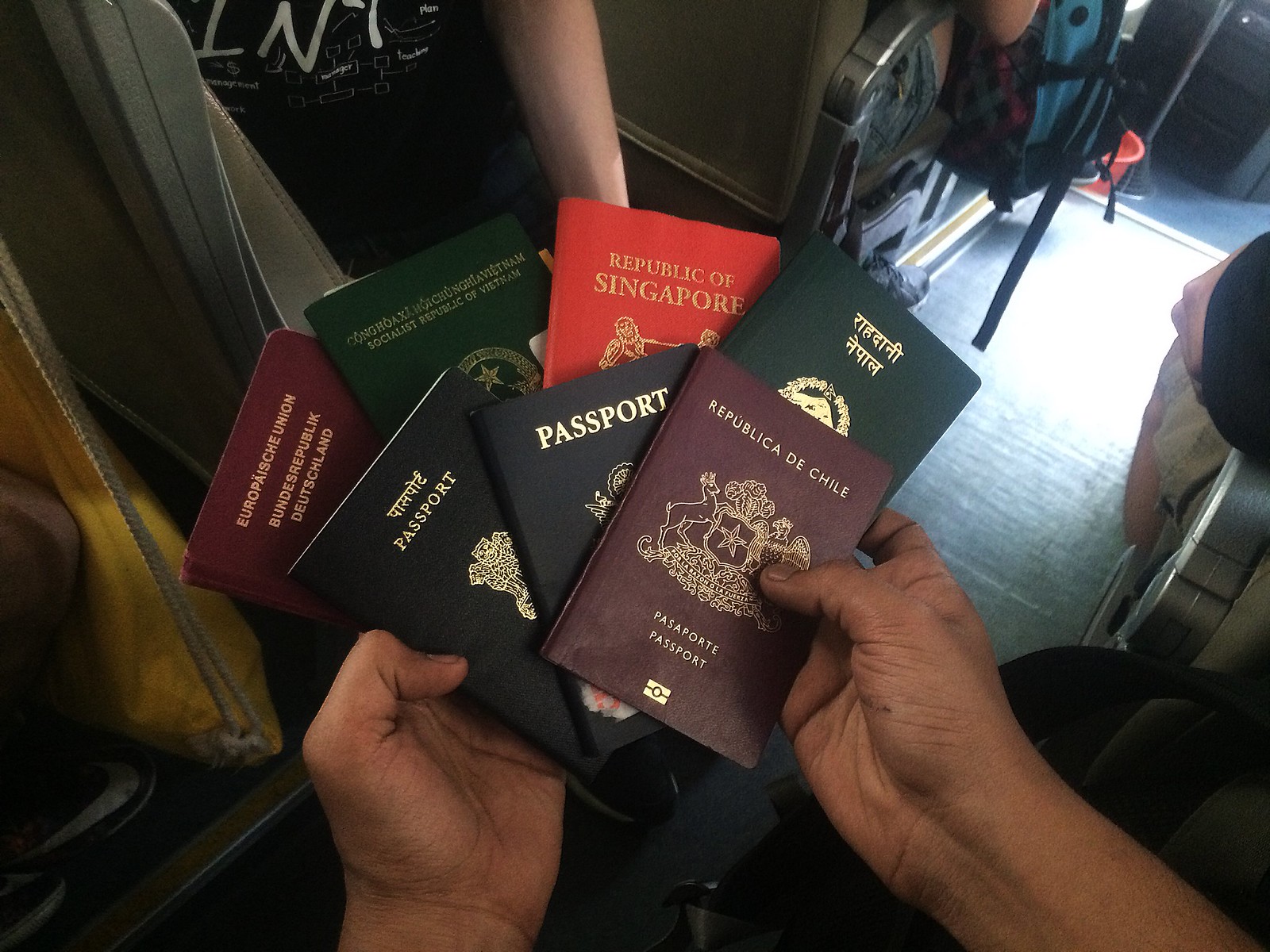The color photograph was taken inside a plane, capturing the interior aisle flanked by tan leather seats with metal handles. The black aisle floor leads to the background of the image, which shows a seated person clutching a blue backpack. At the forefront, a man with dark skin holds out his hands, palms up, displaying seven passports in a fanned-out arrangement. In the top row, there's a maroon passport labeled "Republic of Chile," followed by a dark green passport, a red one marked "Republic of Singapore," and another green passport. The bottom row features a black passport simply labeled "passport," a blue passport, and another maroon passport. Another human arm is visible to the side, clad in a black t-shirt with white writing. The varied languages on the passports hint at a diverse group of travelers.